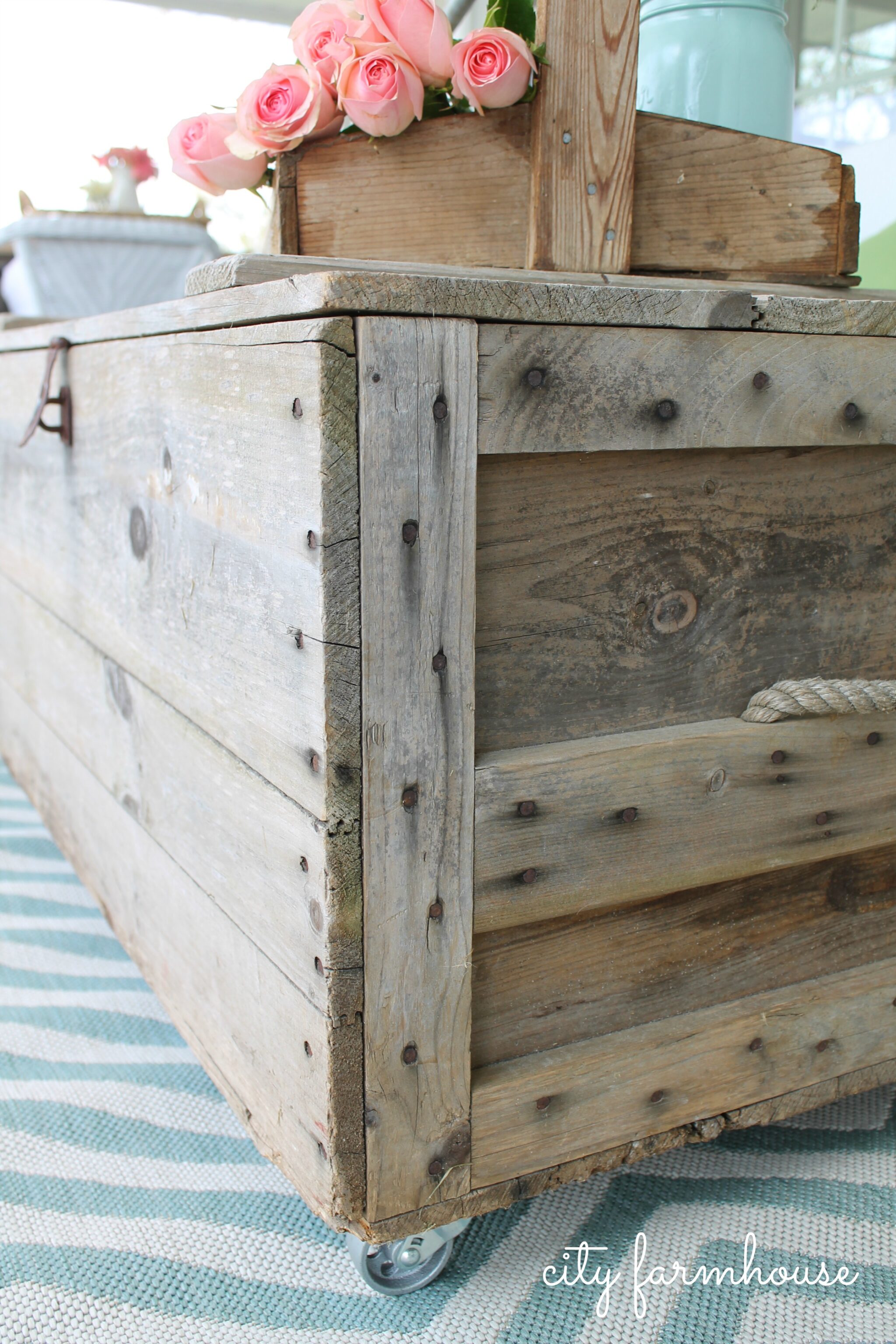This is a detailed color photograph featuring a large, unpainted wooden crate with light-colored wood, complete with knot holes and dark areas, resting on caster wheels. The crate features a rope handle on its right side and an old rusty locking mechanism, suitable for attaching a lock, though currently, no lock is present and the latch hangs over the U-shaped lock component. The crate is angled and positioned atop a teal and white chevron-patterned rug. Sitting on top of the crate is a smaller wooden box with a handle, holding a vibrant arrangement of light pink roses, facing the viewer. In the blurred background, there is a white box or crate also filled with additional flowers, possibly red roses, in what appears to be a vase. The bottom right corner of the image contains the text "City Farmhouse" in a distinctive white cursive script. The overall setting suggests it is daytime.